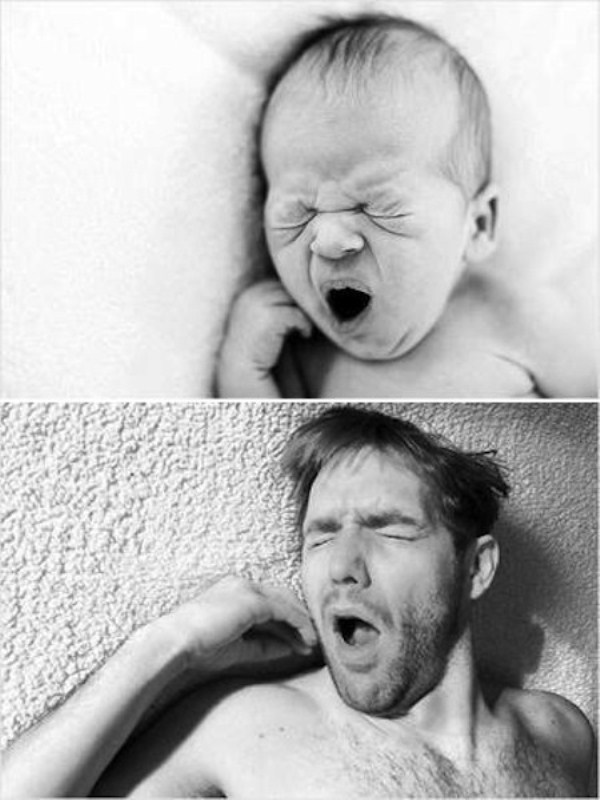The image is a black-and-white photograph featuring two vertically aligned images that present an intriguing juxtaposition. The top photograph captures a recently born infant, likely just a few months old, with very little hair and a scrunched, yawn-like expression. The baby's eyes are closed, and its right hand is gently resting against its right cheek. The infant appears to be lying on a large, fluffy towel or pillow. Below, the lower photograph mirrors the upper one with what seems to be the same individual, now a 25- to 30-year-old man, recreating the exact pose and expression from his infancy. He lies on a textured surface that could be a carpet or towel, with his hair tousled and a few days' growth of beard adorning his face. His right hand replicates the same position against his cheek, and his eyes are closed as he emits a similar yawn-like expression. His bare chest, noticeably hairier than the infant’s, adds to the detailed parallel between the past and present, highlighting an intriguing 30-year time span between the two moments.